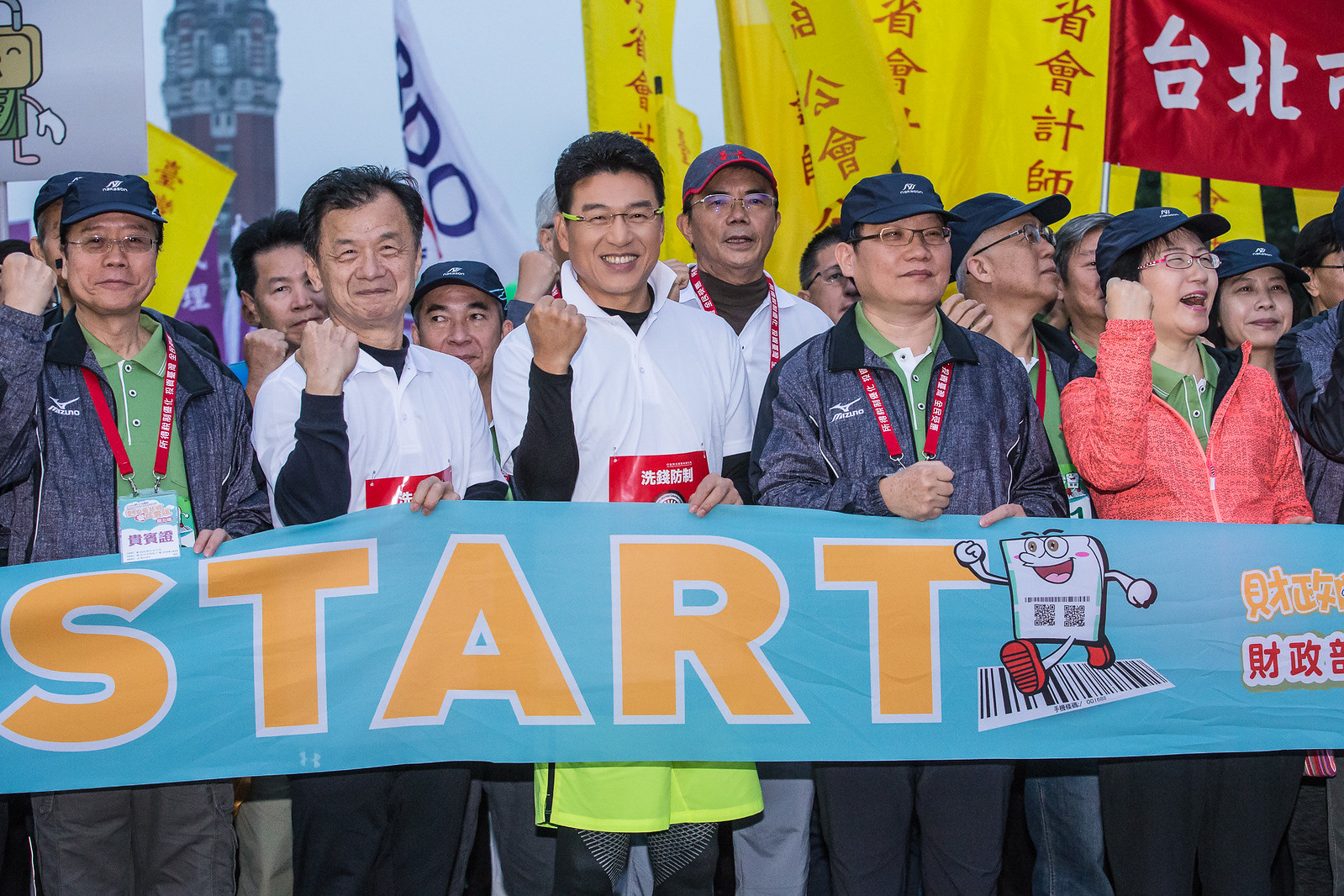In this energetic image, a group of enthusiastic men, many donning baseball hats and wearing name tags or press passes around their necks, stand together with grins on their faces and fists raised in a celebratory gesture. They are gathered behind a blue cloth banner emblazoned with the word "START" in large orange letters. One notable feature of the banner is a playful illustration of a cartoon character resembling a walking notebook or lottery ticket. In the backdrop, there are numerous signs and banners adorned with Asian, likely Chinese, text in red and yellow hues, adding a vibrant cultural context to the scene. This lively gathering appears to mark the commencement of an event, perhaps a marathon or similar activity, given the visual cues and the excitement evident in the crowd's stance and expressions.